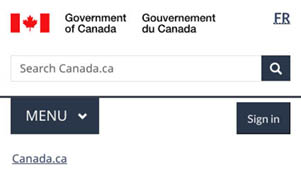This image is a screenshot taken from a mobile phone, displaying the homepage of the Government of Canada's official website. The overall background is white, ensuring a clean and professional appearance. In the upper left-hand corner, there is the prominent Canadian flag, characterized by two vertical red bars flanking a red maple leaf centered on a white square. To the right of the flag, bold black text spells out "Government of Canada," followed by the French translation "Gouvernement du Canada." 

In the upper right-hand corner, underlined letters "FR" signify a language option for French. Directly beneath this heading lies a search bar, featuring a small gray square with a magnifying glass icon. The placeholder text within the search bar reads "Search Canada.ca." Below the search area, a thin black line delineates the interface, accompanied by a black rectangle containing a drop-down menu. To the immediate right, there's a conspicuous black sign-in button.

At the bottom of this section, small gray underlined text reads "Canada.ca," serving as a hyperlink. The remainder of the page appears blank, maintaining the white background and emphasizing the structured layout of the header elements.